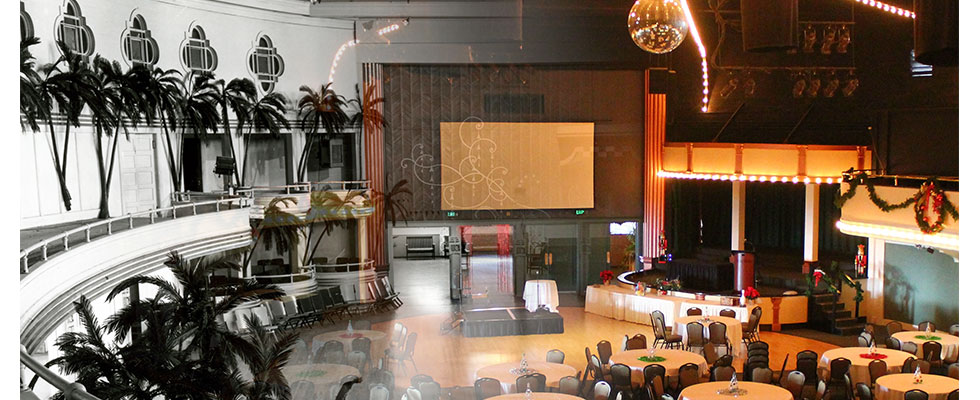The image captures an indoor color photograph of a ballroom or a convention hall, likely set up for a banquet or a concert. The photographer is positioned on an upper balcony, providing a comprehensive view of the scene. On the left side, the photo transitions to black and white, highlighting a standing section with a railing for safety. Adorning the background of the balcony are artificial palm trees arranged in a half-circle formation, with additional palm trees positioned on the floor level below. The wall behind the balcony features four rose-shaped windows and has a gentle curve. A disco ball hangs from the ceiling, along with prominent lighting fixtures and a warm, orangey-toned chandelier.

Toward the center of the image, a stage is set up with a speaking podium and a long, black-draped table. A large rectangular screen or TV is positioned just off to the side of the stage. Decorative elements suggest a Christmas theme, with nutcracker figures on the stage, a large wreath, and garlands draped over the balcony railing to the right. 

In front of the stage, numerous round banquet tables are arranged, each seating about six to eight chairs. The tables feature centerpieces in various colors, such as green and red, and are surrounded by brown chairs. Approximately six or seven tables are visible in the immediate foreground on a tan, wooden dance floor. The overall atmosphere blends festive decorations with elegant architectural details, providing a warm and inviting setting.